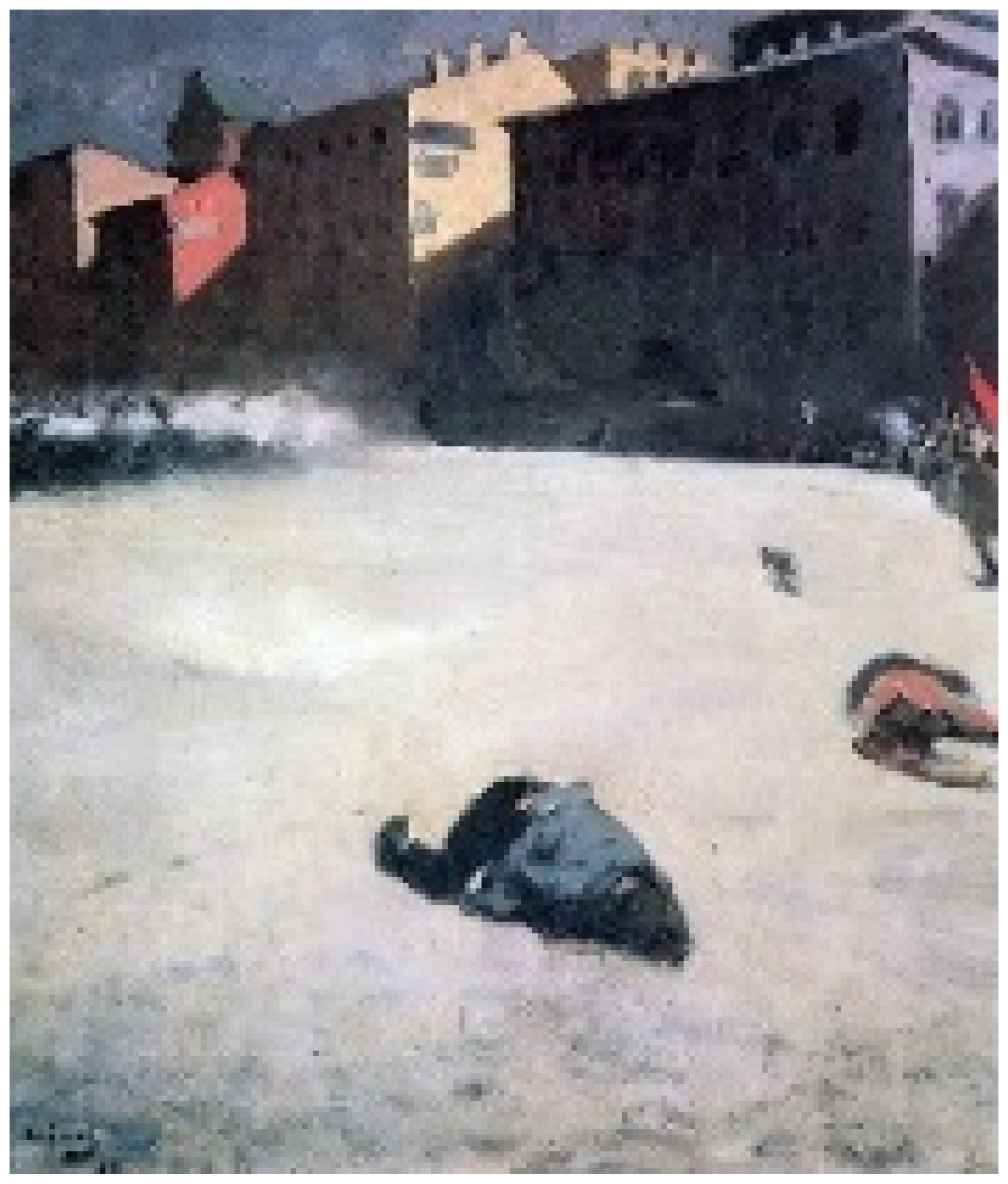The image depicts a blurry and distorted painting with a possible war theme, focusing on two bodies lying in the snow outside. One figure, clad in a blue jacket, and another wearing a red top with long hair, are both positioned on their stomachs approximately three feet apart. The background features a row of multi-storied buildings painted in various colors such as purple, tan, and red. The sky, barely visible, appears as a dark blue, nearly black, and gray hue. On the right-hand side, partially cut off, there are people approaching the scene, suggesting a sense of urgency or aftermath. Despite the foggy and unclear quality of the image, the scene suggests the bleak impact of conflict, with the white ground presumably indicating snow, and the overall setting appearing bright, as if it is daytime.